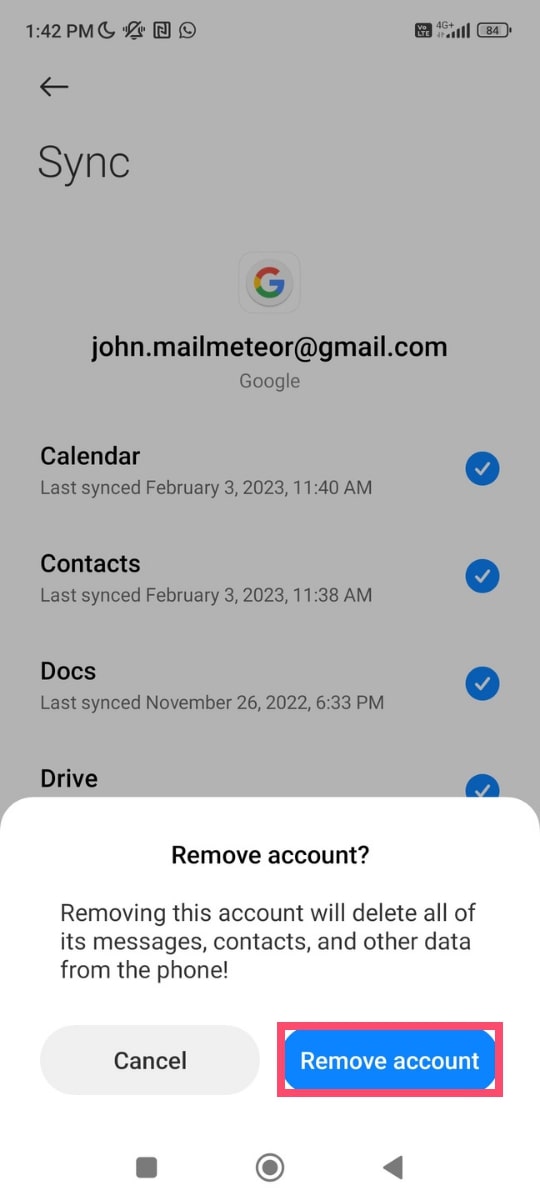The image is a screenshot of an Android device, displaying a Google account sync status and settings. In the top left corner, the screen shows the current time, 1:42 PM, alongside several symbols including a half moon, a bell with a slash through it (indicating notifications are silenced), and a square with a line through it. Additionally, there is an icon resembling a chat bubble with a phone inside it. To the far right of these symbols are network and device status icons: Wi-Fi signal strength, mobile network status, and battery level indicators.

Below these indicators, on the left-hand side, there is a back arrow, and beneath it, the word "Sync" (S-Y-N-C). Centered underneath is the Google icon ("G"), followed by a user's email address, "john.mailmedia@gmail.com", and the word "Google" beneath that.

The main section consists of a list of Google services with their last sync times, each accompanied by a blue circle with a white checkmark. The services and their last sync details are as follows:
1. **Calendar** - Last synced on February 3rd, 2023, at 11:40 AM.
2. **Contacts** - Last synced on February 3rd, 2023, at 11:38 AM.
3. **Docs** - Last synced on November 26th, 2022, at 6:33 PM.
4. **Drive** - The full text for Drive’s last sync status is partially cut off, but a blue circle with a checkmark can be seen.

The bottom section contains an option to "Remove account" with a detailed warning stating, "Removing this account will delete all of its messages, contacts, and other data from the phone!" Below this, there are two buttons: "Cancel" on the left and "Remove account" on the right, the latter highlighted with a red rectangular outline.

At the very bottom, there is a filled gray square with a gray circle inside, and another filled circle in the middle of that. Finally, there is an arrow pointing to the left.